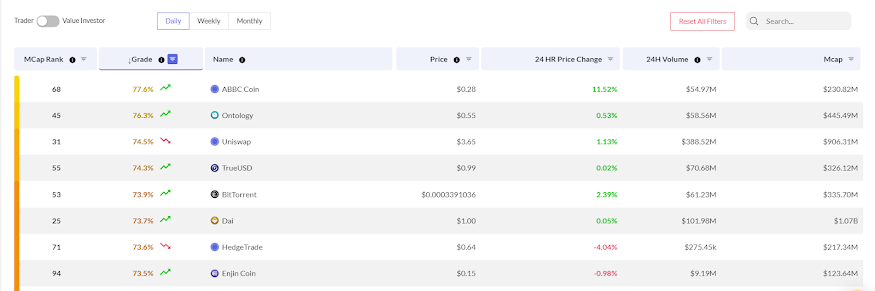This screenshot showcases a section of an interface from an unidentified source, likely related to cryptocurrency trading and investments. The top header displays options and filters with a primary title "Trader" followed by a secondary title "Virtue Investor". Below this header, a toggle switch is set to "Daily" mode, with additional filter options for Weekly, Monthly, Reset All Filters, and a Search function. The information is categorized into columns labelled MCAP Rank, Grade, Name, Price, 24-Hour Price Change, 24-Hour Volume, and MCAP.

Each row presents detailed information for specific cryptocurrencies:

1. **Rank 68** - **ABBC Coin**
   - **Grade:** 77.6% up
   - **Price:** $0.28
   - **24-Hour Price Change:** 11.52%
   - **24-Hour Volume:** $54.97M
   - **Market Capitalization (MCAP):** $230.82M

2. **Rank 45** - **Ontology**
   - **Grade:** 76.3% up
   - **Price:** $0.55
   - **24-Hour Price Change:** 0.53%
   - **24-Hour Volume:** $58.56M
   - **Market Capitalization (MCAP):** $445.49M

3. **Rank 31** - **Uniswap**
   - **Grade:** 74.5% down
   - **Price:** $3.65
   - **24-Hour Price Change:** 1.13%
   - **24-Hour Volume:** $388.52M
   - **Market Capitalization (MCAP):** $906.31M

4. **Rank 55** - **TrueUSD**
   - **Grade:** 74.3% up
   - **Price:** $0.99
   - **24-Hour Price Change:** 0.02%
   - **24-Hour Volume:** $70.68M
   - **Market Capitalization (MCAP):** $326.12M

5. **Rank 53** - **BitTorrent**
   - **Grade:** 73.9% up
   - **Price:** $0.0003391036
   - **24-Hour Price Change:** 2.39%
   - **24-Hour Volume:** $61.23M
   - **Market Capitalization (MCAP):** $335.70M

6. **Rank 25** - **DAI**
   - **Grade:** 73.7% up
   - **Price:** $1.00
   - **24-Hour Price Change:** 0.05%
   - **24-Hour Volume:** $101.98M
   - **Market Capitalization (MCAP):** $1.07B

7. **Rank 71** - **Hedgetrade**
   - **Grade:** 73.6% down
   - **Price:** $0.64
   - **24-Hour Price Change:** -4.04%
   - **24-Hour Volume:** $275.45K
   - **Market Capitalization (MCAP):** $13.34M

8. **Rank 94** - **EngineCoin**
   - **Grade:** 73.5% up
   - **Price:** $0.15
   - **24-Hour Price Change:** -0.98%
   - **24-Hour Volume:** $9.19M
   - **Market Capitalization (MCAP):** $123.64M

This summary delivers a comprehensive view of the cryptocurrency market performance metrics as listed in the interface, highlighting the ranks, trading grades, prices, volume changes, and market capitalizations.